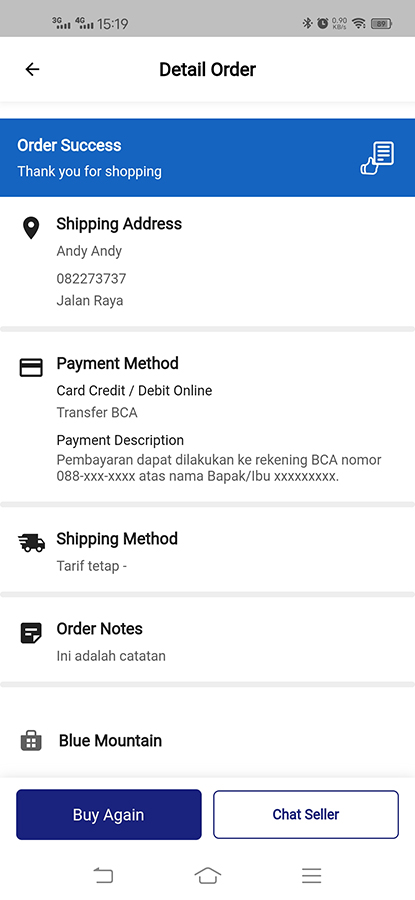Screenshot of a mobile website displayed on an Android device. The top status bar shows multiple signals with full strength, including a 3G signal, a 4G signal, Wi-Fi, and Bluetooth. The time is 15:19, the device has 89% battery remaining, and the network speed is 0.9 kilobytes per second. The screen displays an order confirmation page titled "Detail Order," indicating a successful transaction with the message, "Order Success. Thank you for shopping," accompanied by a thumbs-up icon within a blue rectangle.

The shipping address is listed as "Andy, Andy 08227-3737 Jalan Raya," and the payment method used is a credit card/debit card via online transfer through BCA. The payment description includes "Pemba Raya Depat Dilakan Kekekan BCA Nomor 088," and the shipping method is "Tariff Tepap." Order notes mention "Ini Adala Katatan" and reference "Blue Mountain" at the bottom of the screen. There are two actionable buttons at the bottom: a blue "Buy Again" button on the left and a white "Chat Seller" button on the right.